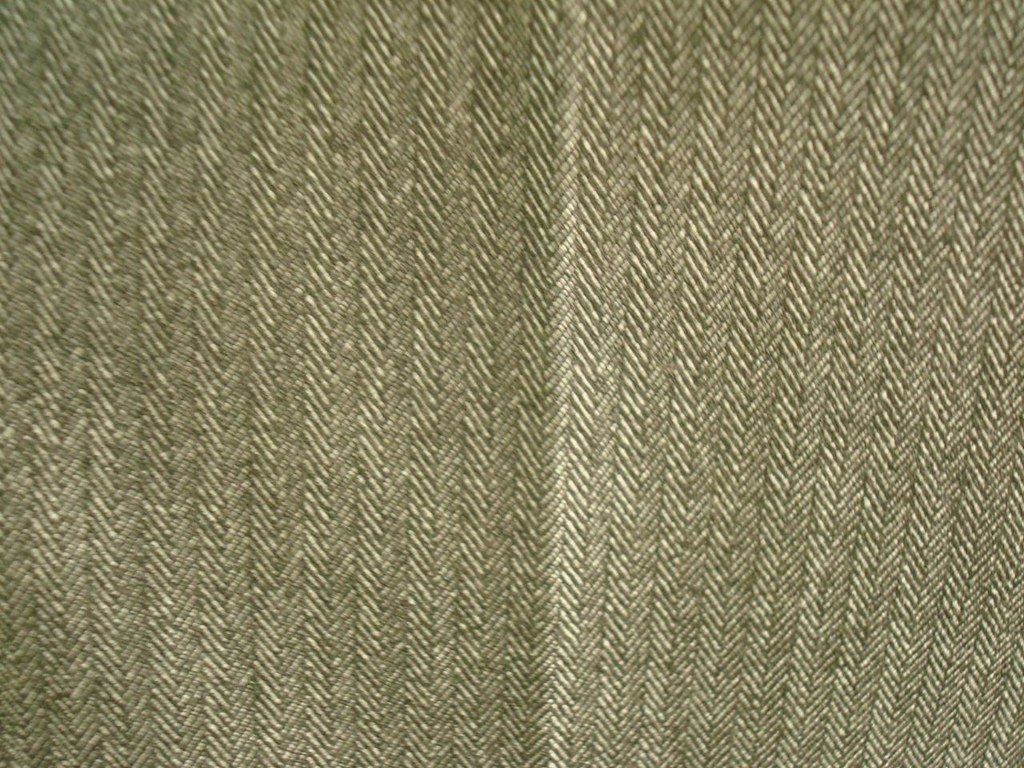The image depicts a close-up rectangle of fabric, potentially from a curtain, pant leg, or rug, exhibiting a detailed pattern. This pattern primarily consists of vertical stripes in shades of green, brown, tan, and gray, with alternating lines of green and white. There are also diagonal stripes that intersect the vertical ones, adding to the intricate design. A prominent crease runs down the center of the fabric, protruding slightly toward the viewer and highlighted by a brighter area. The top left portion of the photograph is somewhat blurry, while the center and especially the right side are in sharper focus. The fabric's texture and pattern are meticulously detailed, featuring vertical columns of fabric with lines that extend from the top to the bottom and from left to right.